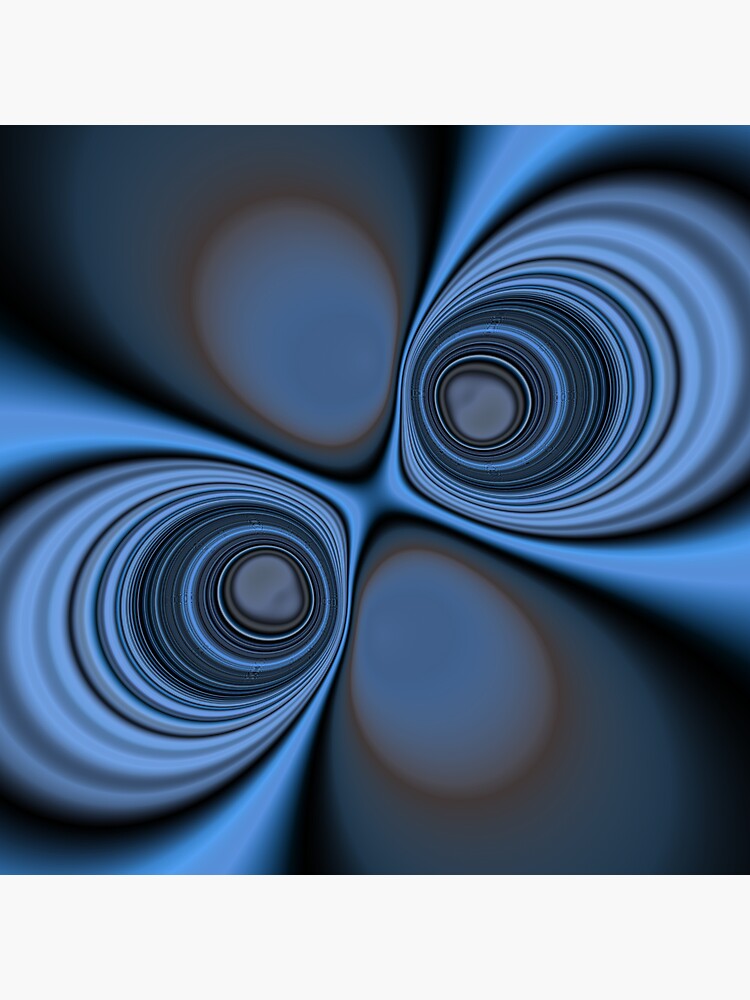This abstract artwork presents a striking array of colored circles and ovals set against a dark background, creating a mirrored and symmetrical composition. The central motif features large, eye-like shapes with a complex, marbled swirl transitioning from light to dark blue. These shapes occupy the top left and bottom right corners, each encircled by smaller, tan and blue orbs. The top right and bottom left areas mirror each other with clusters of smaller circles in black, white, and various shades of blue, enhancing the overall symmetry. Resembling alien eyes, the intricate web of colors—gray, brown, blue, and black—creates an engaging, otherworldly visual experience, alluding to the artist's abstract and imaginative vision.